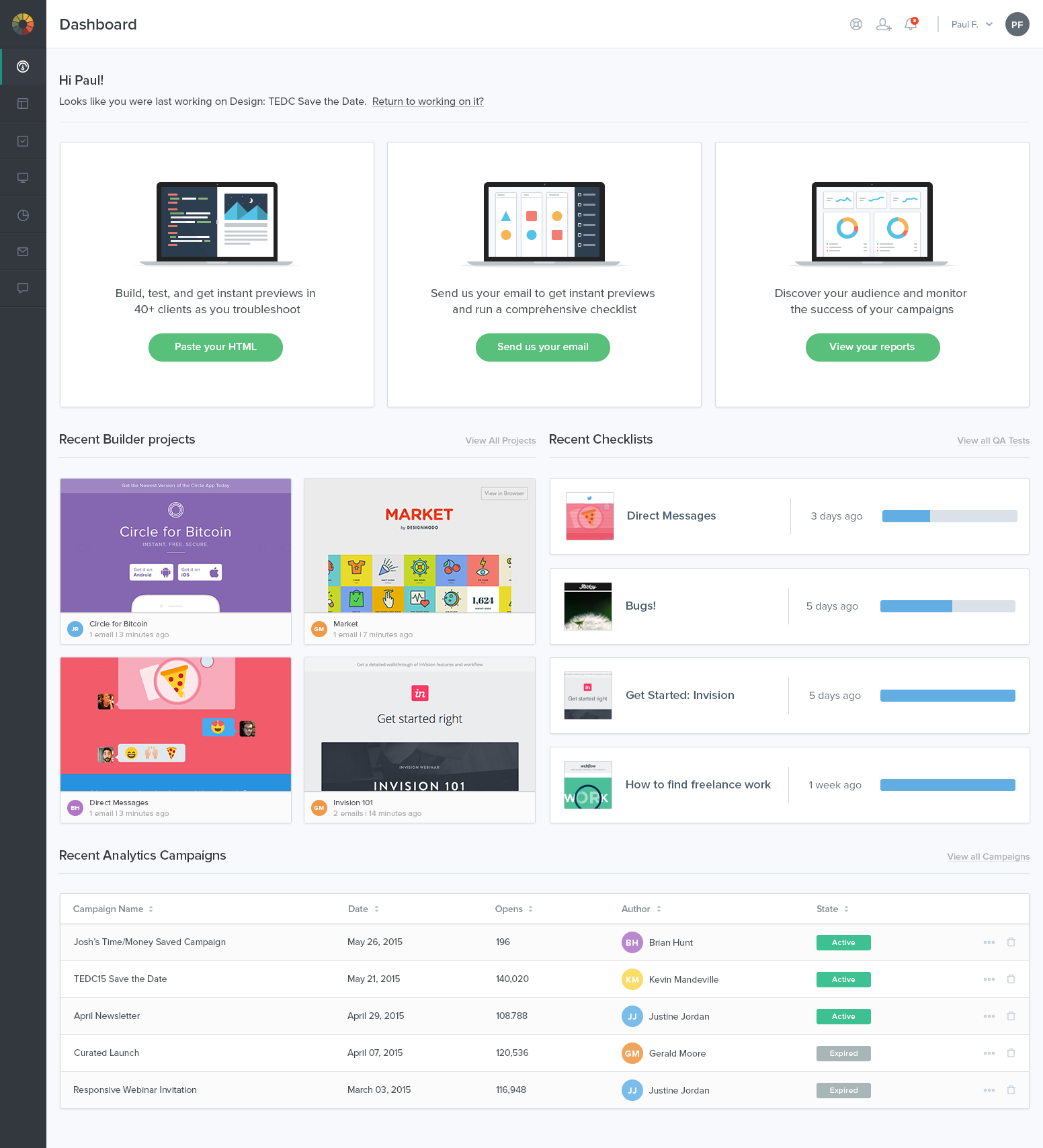The image displays a user interface with numerous elements, starting with a long, dark grey rectangle on the left-hand side. At its top, there is a color wheel followed by a white circle containing indiscernible icons and some grey symbols. To the right of the color wheel, the word "Dashboard" is prominently displayed. Adjacent to this, there is an outlined grey circle with unclear contents, a person symbol, a bell with a red circle indicating a notification, some illegible words, a downward-pointing arrow, and a grey circle with the initials "PF."

Below this section, it greets the user with "Hi Paul," followed by more unreadable text. Three white rectangles line the interface, each displaying a laptop with various content: the first rectangle shows numerous words to the left and a picture of mountains with text on the right; the second contains different colored shapes with a line of text on the right; the third showcases charts in blue, yellow, and orange hues. At the bottom of these rectangles are bars labeled "Place your HTML," "Send us your email," and "View your records."

The lower section features headers, such as "Recent Building Builder Projects" and "Recent Checklists," with minuscule, unreadable text beneath them. A purple box captioned "Circle for Bitcoin" is followed by a layered purple circle with a dark purple inside and a legged circle bar with text that is too tiny to read. To the right are two white rectangles with purple symbols and left-aligned writing, all atop a white bar.

Further down, a grey rectangle labeled "Market" appears at the top, followed by unreadable text and various multi-colored square symbols. Adjacent to this, on the left, is a pink rectangle with a light pink overlay featuring a circle containing a pizza, followed by a blue rectangle with a happy face and heart eyes, a vague black symbol, and indiscernible icons at the bottom, next to a blue bar.

The next portion contains a grey rectangle with a red square with text "Get Started" and a black rectangle with tiny words, leading into other cropped words. To the right are white rectangles with pictures labeled "Direct Messages," "Bugs," "Get started in Vision," and "How to Find Freelance Work." More unreadable writing appears on the right with bars in blue and grey, varying in length, with two bars entirely blue. Below that, "Recent Analytics Campaigns" is mentioned above a white rectangle covered in grey lines and minuscule words. Colored circles (purple, yellow, orange, and blue) with text inside are followed by three green rectangles with small text and two grey rectangles with similarly unreadable writing.